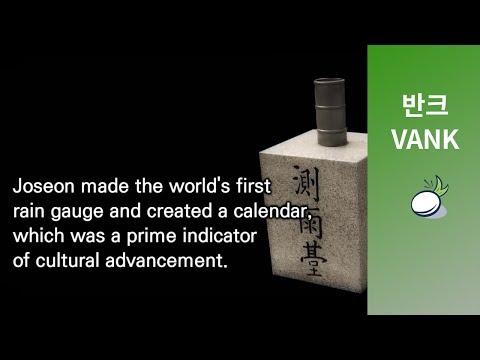The image presents a visually compelling and informative composition against a solid black background. On the left side, a paragraph in white text reads: "Joseon made the world's first rain gauge and created a calendar, which was a prime indicator of cultural advancement." This text is left-aligned and serves as an introduction to the main subject on the right side of the image. 

Prominently displayed is a vertically positioned ring gauge, which rests upon a marble-like rectangular stone base. Emerging from the center of this stone structure is a circular metal probe, resembling a gray pipe or chimney. The front surface of the stone base features three vertically arranged Chinese characters, 七宇台, inscribed in black. 

To the far right of the image is a green rectangular area, resembling a digital display, which contains two white symbols and the word "VANK" in all caps. Below this text, a circular white object with two green leaves protruding from the top is depicted, reminiscent of an egg or possibly an onion, providing a modern contrast to the ancient instrument showcased.